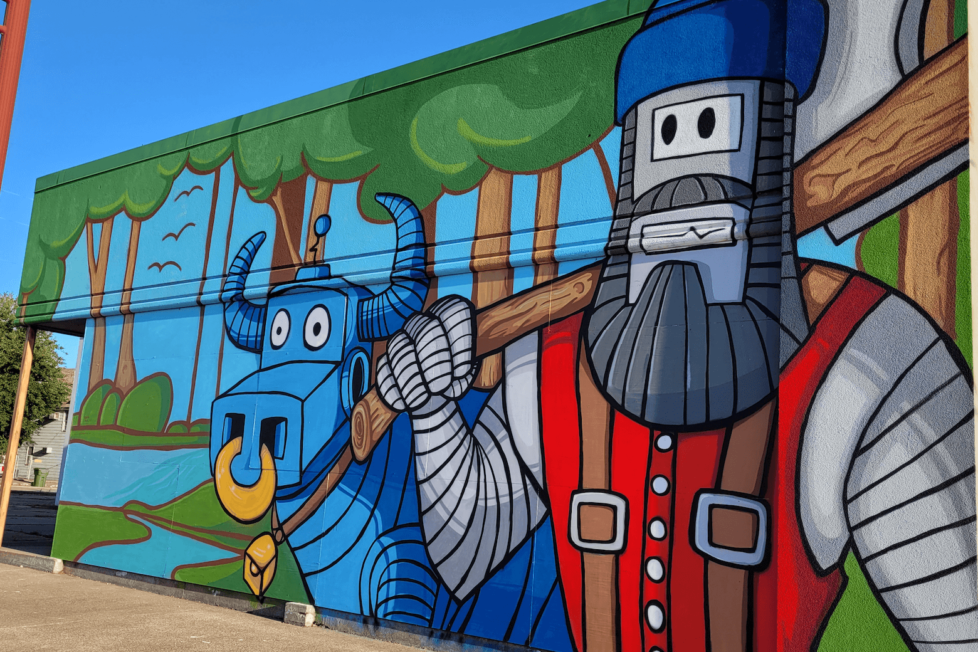The photograph, taken outdoors during the daytime, captures a highly detailed mural painted on the side of a low warehouse-style building, likely located in a parking lot. The mural depicts a vibrant, whimsical forest scene featuring two distinctive, cartoony characters: Paul Bunyan and Babe the Blue Ox. This modern rendition of the famed duo showcases them with a robotic, Futurama-esque twist. Paul Bunyan, adorned in a blue knit cap, a red shirt, and brown leather suspenders, carries a wooden axe over his shoulder. His metal-like appearance includes a robotic face. Beside him stands Babe the Blue Ox, also rendered in a metallic, robotic style. Babe sports a blue coat, a golden nose ring, an antenna on top of his head, and a gold bell dangling from a brown strap around his neck. The mural's background is rich with natural elements, featuring trees with brown trunks and green leaves, a serene river, lush green grass, and various bushes. The scene extends to show mural birds flying in the sky, completing the detailed and colorful narrative painted on the building's side.